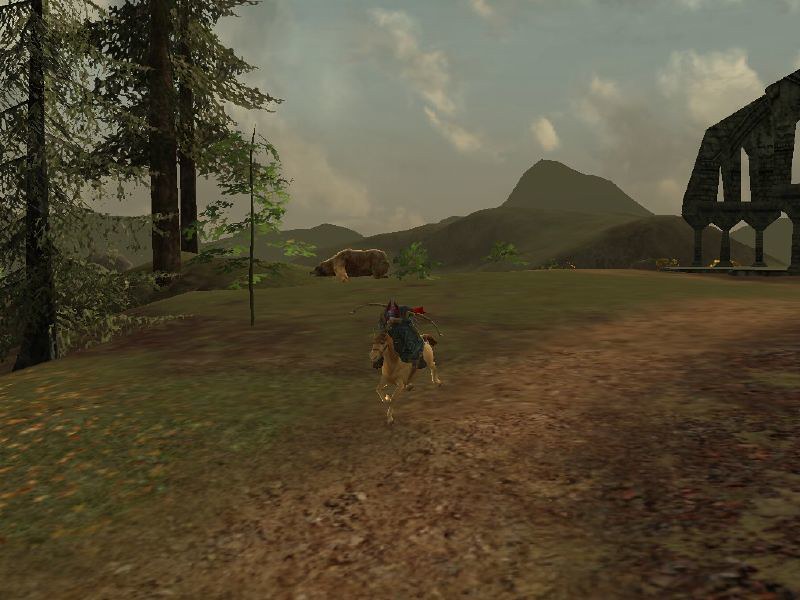This image, possibly a digital artwork or painting resembling a scene from a video game, portrays an expansive outdoor landscape filled with various natural and structural elements. Dominating the background is a range of mountains, with one notably sharp peak piercing the sky. The sky above is a light blue, dotted with large, billowing white clouds, adding depth and a sense of serenity to the composition.

On the left side of the image stand towering trees with impressively wide trunks, their tops extending beyond the frame's edge, emphasizing their great height. Beneath the trees stretches a vast, verdant field, interspersed with patches of light brown dirt or possibly fallen leaves forming a meandering path through the greenery.

Central to the scene is a striking figure: a horse with a rider, who appears to be brandishing a sword, suggesting a moment of action or adventure. The mid-ground features a mysterious creature that resembles a hippopotamus, adding an element of fantasy or intrigue to the setting. Scattered throughout the landscape are smaller trees or dense bushes, contributing to the diverse vegetation of the field.

Off to the right side of the image stands an enigmatic structure. This building, supported by four sturdy pillars, has an open, almost skeletal appearance with its black frame and slit-like windows that allow the sky to be visible through them, creating an eerie or unfinished look.

Together, these elements weave a rich and dynamic scene, replete with natural beauty, subtle mysteries, and a sense of impending narrative, inviting viewers to step into this fantastical world and explore its depths.